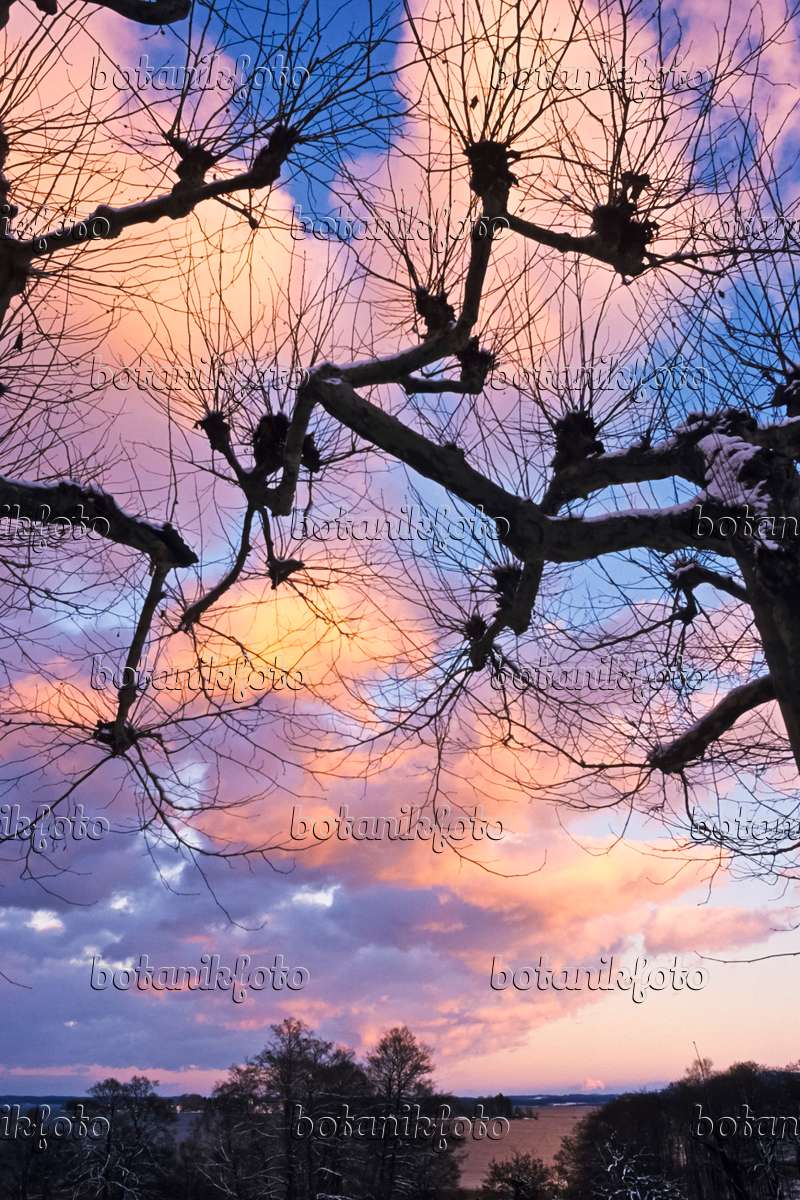The photograph captures a dramatic outdoor scene, dominated by a vibrant and colorful sky filled with pink, orange, and blue hues indicative of either sunrise or sunset. The sky is partially covered by clouds tinged with these colors, creating a serene yet dynamic atmosphere. Black or dark gray branches of a spiky tree stretch across the photo, resembling a spider's web and casting intricate shadows. The base of this tree is positioned on the right side, with its branches fanning out to the left. Below, the darker silhouettes of trees and bushes appear in shadow, some showing leaves. A body of water, possibly a river or lake, is faintly visible in the background at the bottom of the image. Throughout the photograph, a watermark reading "Botanique Photo" is overlaid multiple times, ensuring the image's protection against unauthorized use.